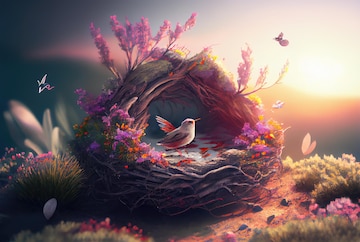In the center of this highly detailed color illustration, a rounded, ornate bird nest is depicted, sitting amidst a lush garden setting. The basket-shaped nest, crafted from interwoven twigs, features an elegant arched covering on top, possibly hinting at a fantasy theme. The nest is adorned with vibrant flowers: delicate pink and orange blooms flank the left and right sides of the entrance, while longer pink flowers cascade from the back and gracefully arch over the top.

Inside the nest, a small bird with a cream-colored body and wings that blend dark red at the base into white at the tips, is positioned facing to the right, looking slightly upward. Surrounding the nest is a field of soft grass interspersed with additional pink flowers, enriching the foreground.

To the right of the nest, the illustration captures a serene sunset, with a warm lemon yellow hue illuminating the horizon. Above and below the sunset, several butterflies can be seen fluttering. On the top left, a hummingbird hovers, adding to the dynamic nature of the scene.

The sky in the background, despite the day setting suggested by the sunlight, is artistically blurred and somewhat darker, enhancing the focus on the vivid details of the foreground elements. This intricately depicted scene is rich with colors and textures, merging the realms of nature and fantasy in a strikingly beautiful composition.